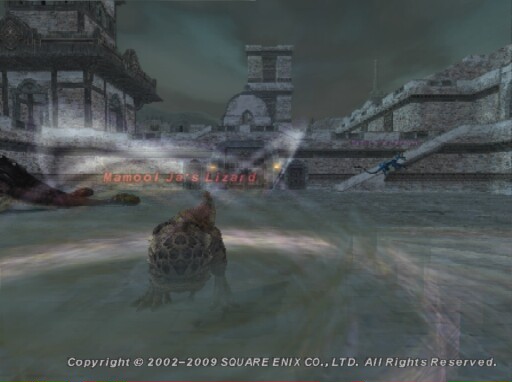The image appears to be a detailed screenshot from a video game, highlighted by an intricate setting and specific features. At the forefront is a shallow body of water, with a turtle-like creature emerging, its shell and head distinctly visible. This scene is encased within a stone-built village stretching horizontally from left to right. The village showcases weathered stone huts and structures, with notable stone stairs adding to its ancient ambiance. Above the aquatic creature, the orange text reads "Mamool Jars Lizard," while the backdrop features large, castle-like structures in varying shades of gray and black, reflecting an old and imposing architecture. The skyline presents a somber, dark grey to greenish-blue hue, encapsulating a moody atmosphere. The bottom of the image is marked with a white text watermark stating "Copyright 2002-2009, Square Enix Co. Ltd. All Rights Reserved." This comprehensive scene blends elements of both fantasy and medieval design, reinforcing its video game origin.